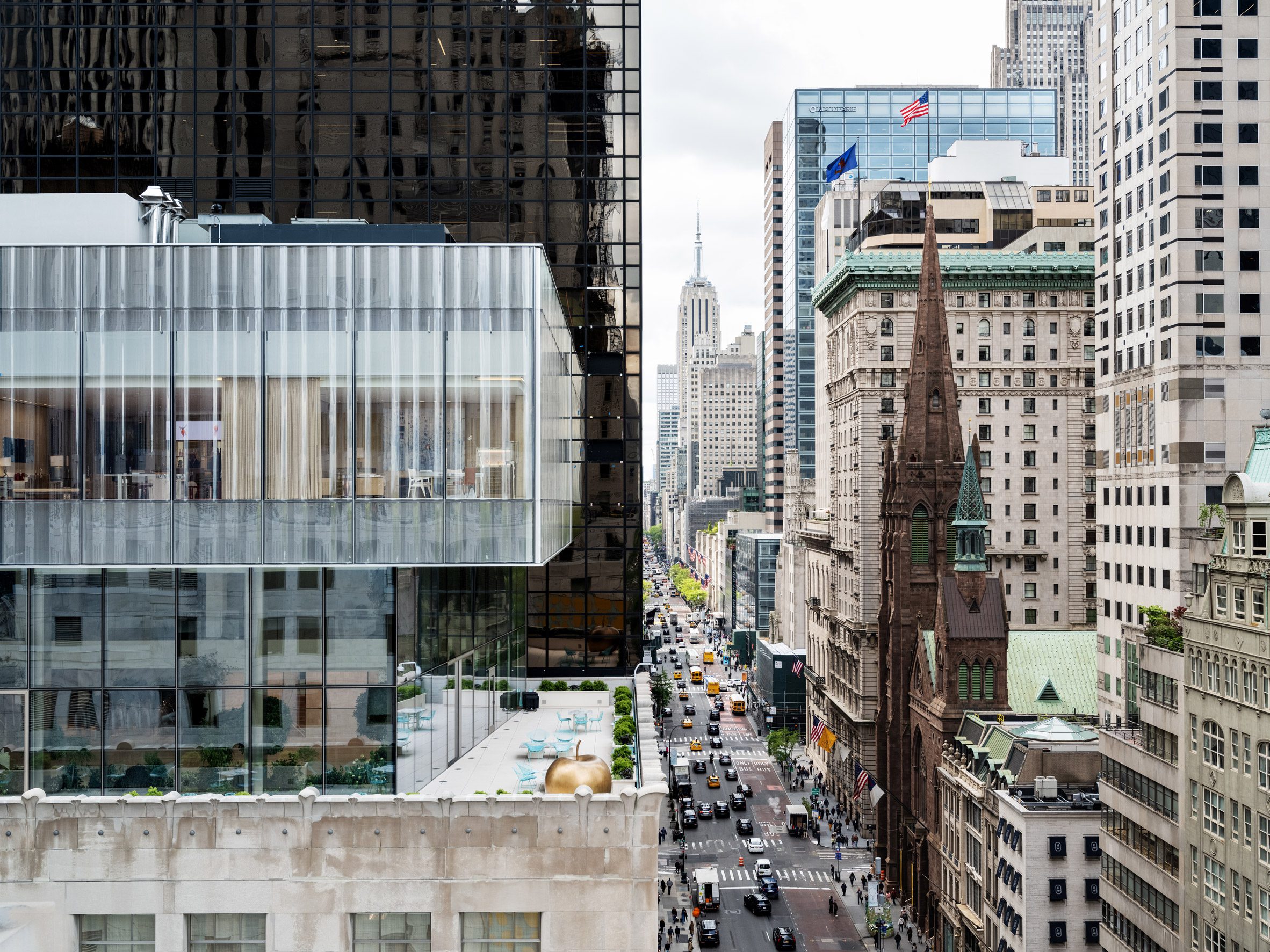This compelling cityscape photograph, likely taken from an elevated viewpoint within a building, showcases a bustling city street framed by imposing high-rise structures, suggesting a vibrant urban scene that might be New York City. Central to the composition, a stark visual line is created by a dark glass skyscraper juxtaposed against the edge of a balcony from an adjacent building, evoking the illusion of two separate photographs seamlessly merged. Down the congested, likely one-way street, a distant, towering structure punctuates the skyline amidst a sea of traffic. In the mid-ground, a dark, brownish building adorned with possible brass detailing rises, distinguished by a turret topped with an American flag, hinting at a historic or ecclesiastical role. The building closest to the photographer is a modern office edifice with expansive glass windows, featuring a balcony festooned with plants and seating, adding a touch of greenery to the urban tableau. The scene is captured in daylight under a cloudy sky, emphasizing the dynamic yet introspective nature of city life, devoid of visible inhabitants but bustling with vehicular activity.